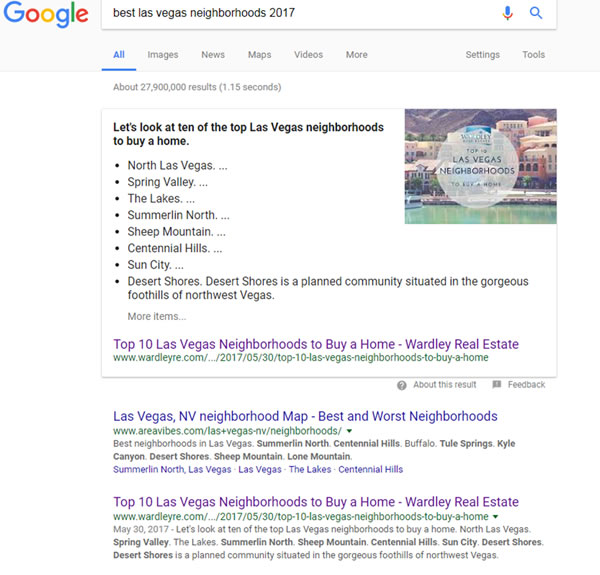A Google search results page is displayed, with the familiar Google logo at the top left, showcasing its multicolored lettering. The search query entered is "best Las Vegas neighborhoods in 2017." On the far right of the search bar are the search icon and a microphone icon, enabling voice search.

Just below the search bar, there are various navigational options including "All," "Images," "News," "Maps," "Videos," "More," along with "Settings" and "Tools." The "All" category is currently selected, revealing approximately 27,900,000 results which were generated in 1.15 seconds.

The first result is a non-sponsored link titled "Let's look at 10 of the top Las Vegas neighborhoods to buy a home." It lists several neighborhoods such as North Las Vegas, Spring Valley, The Lakes, Summerlin North, Sheep Mountain, Centennial Hills, Sun City, and Desert Shores. Desert Shores is described as a planned community located in the picturesque foothills of Northwest Vegas.

Next, there is an option to view more items via a link to "Top 10 Las Vegas neighborhoods to buy a home," sponsored by Wardley Real Estate. This link appears in light purple, indicating it has been visited before. Below this is a blue link titled "Las Vegas Nevada Neighborhood Map: Best and Worst Neighborhoods," signifying it has not been clicked on. Another purple link, suggesting prior visitation, is also displayed below, titled "Top 10 Las Vegas neighborhoods to buy a home," again sponsored by Wardley Real Estate.